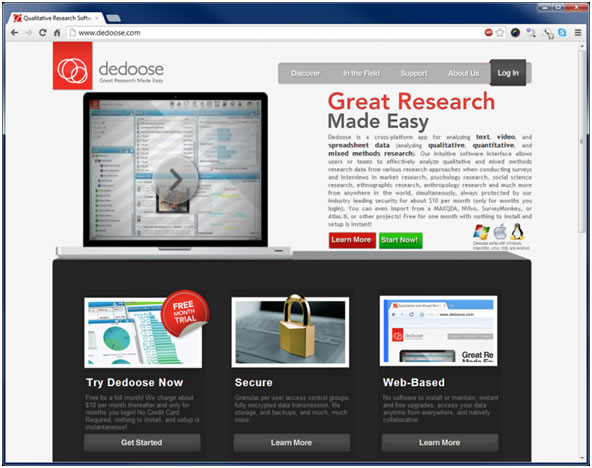The desktop application screenshot depicts the Chrome browser accessing the website www.deduce.com, which is a qualitative research software platform. At the top left of the browser, highlighted by the standard Chrome interface, the site’s address is visible. Deduce's logo, located at the top left of the webpage, consists of multiple overlapping circles against a red background. The website itself predominantly uses a white background for a clean and professional appearance.

Beneath the company's name, the slogan "Great Research Made Easy" is prominently displayed. A central feature of the page is a screenshot of a MacBook Pro with a play button, likely showcasing a demo of the software's capabilities.

To the right, the navigation bar includes several tabs with a gray background labeled as "Discover," "In the Field," "Support," "About Us," and a prominently highlighted "Login" tab. Below the slogan, the text reads "Great Research" in red, followed by "Made Easy" in darker gray. A red "Learn More" button and a green "Start Now" button are positioned directly beneath the slogan.

To the right of these buttons, icons indicate that the software is compatible with Windows, Apple, and Linux operating systems. Lower on the page, additional sections provide shortcuts to getting started with the platform, detailed security information, and web-based features. These sections are depicted on a predominantly black background, emphasizing their importance and accessibility options.